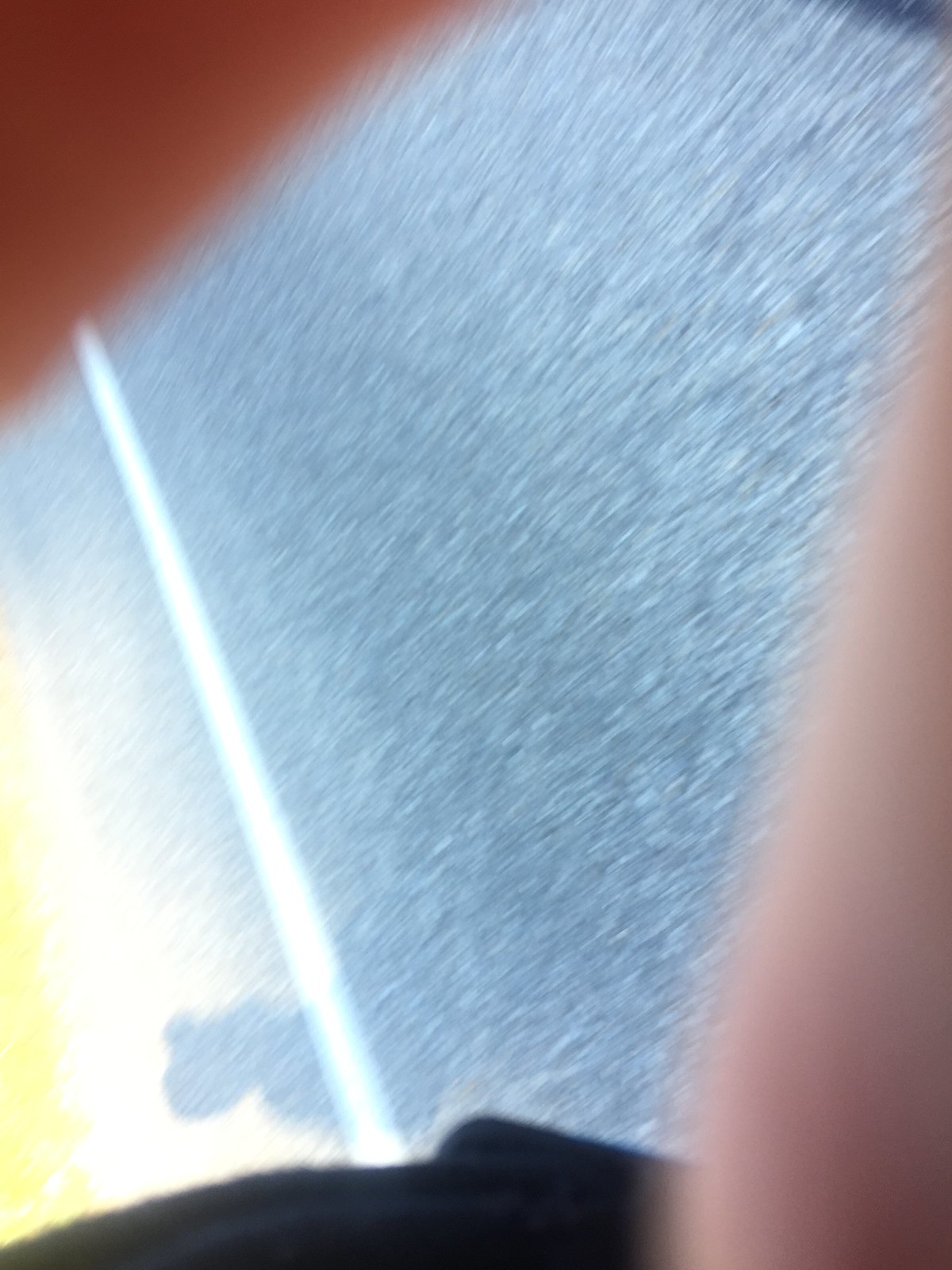The image captures a close-up view of an asphalt ground, peppered with white specks throughout. A long, distinct white line runs vertically on the left side, adjacent to a yellow line at the far left edge. Shadows cast on the ground create additional texture. The bottom right and top of the image are partially obscured by blurry fingers covering the lens, providing an interesting, albeit unintended, frame around the scene. The overall effect gives a sense of immediacy and unfiltered realism.